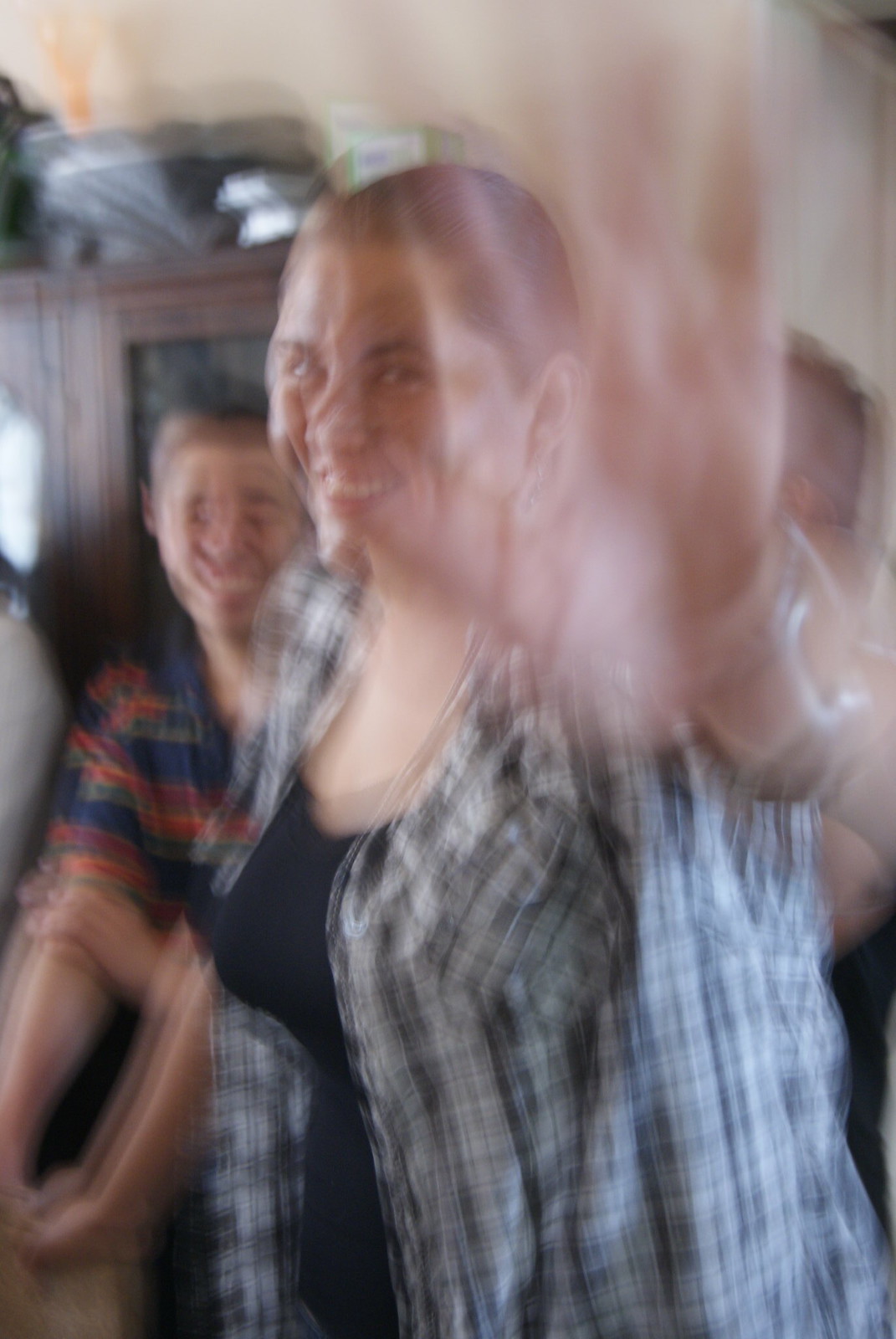The photograph is a vertically-oriented, unintentionally blurry image captured indoors. The blurriness seems to be caused by movement from the subjects in the picture, rather than any artistic intent to focus on a specific area. In the background, there is a large, brown chest of drawers with various items piled on top of it.

At least three people appear in the photograph, including both males and females. The person in the foreground is a female wearing a black tank top with a short-sleeved plaid shirt layered over it. She has very short, buzzed hair and her raised hand contributes to the blurriness. Behind her, there's a boy in an orange and blue striped collared shirt. The details of the third person are less clear, as they are obscured and further back in the frame. The overall scene gives the impression of candid interaction within a home setting.